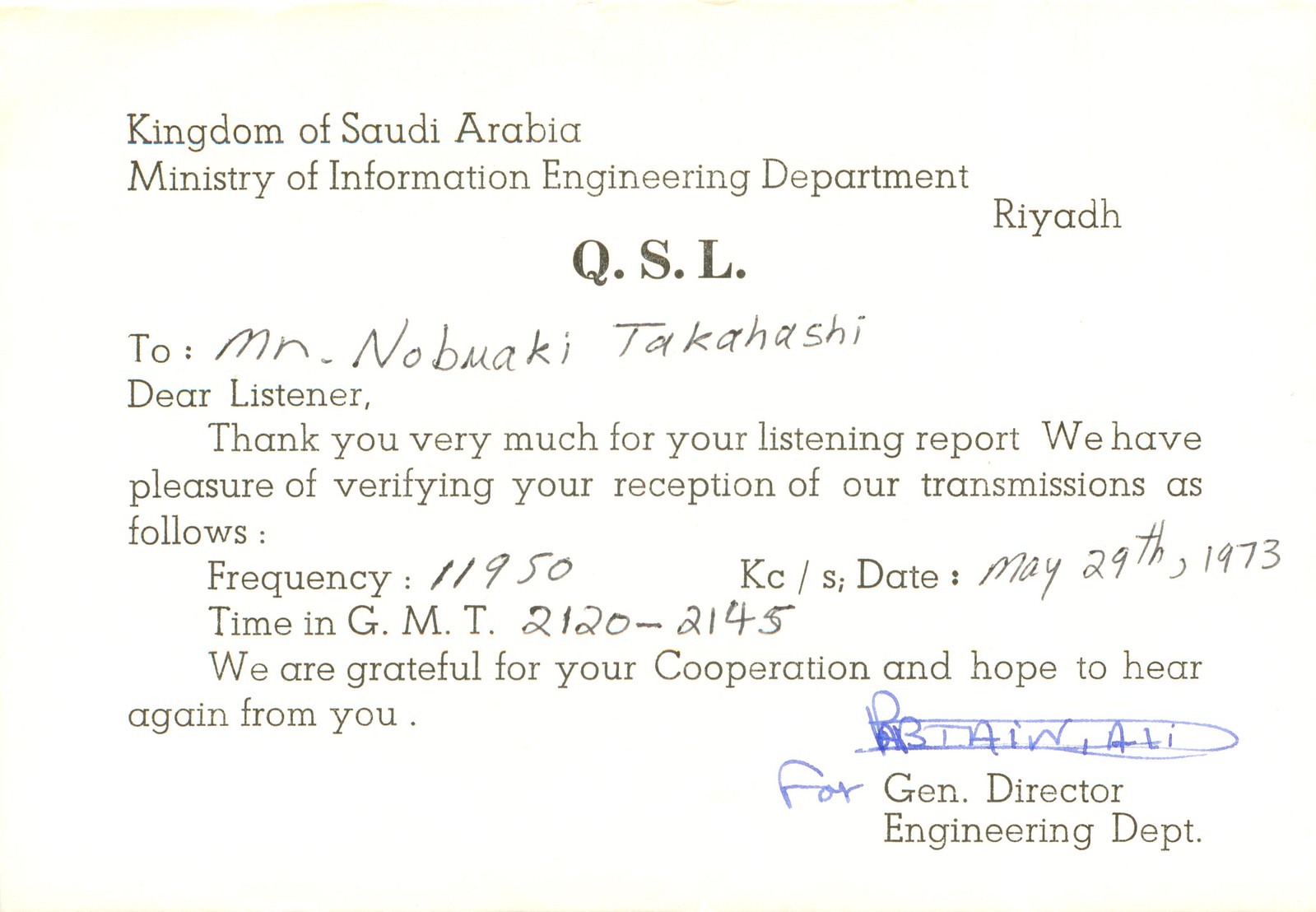The image depicts a typed document on a white background. At the top left in bold letters, it reads "Kingdom of Saudi Arabia, Ministry of Information, Engineering Department." To the right, it has "Riyadh" in uppercase letters. Centered below this header in large black font, the document features "QSL." The text is addressed to "Mr. Nomaki Takashi," with "Dear listener" following in a typed format. The letter thanks Mr. Takashi for his listening report and verifies the reception of the transmission on a frequency of 11950 kHz. The date and time of the reception are noted as "May 29th, 1973," from "GMT 2120-2145." Additionally, the letter expresses gratitude for Mr. Takashi's cooperation and hopes to hear from him again. It is signed by the "General Director, Engineering Department." There is also some crossed-out blue writing above the director’s signature, with only partial letters legible.